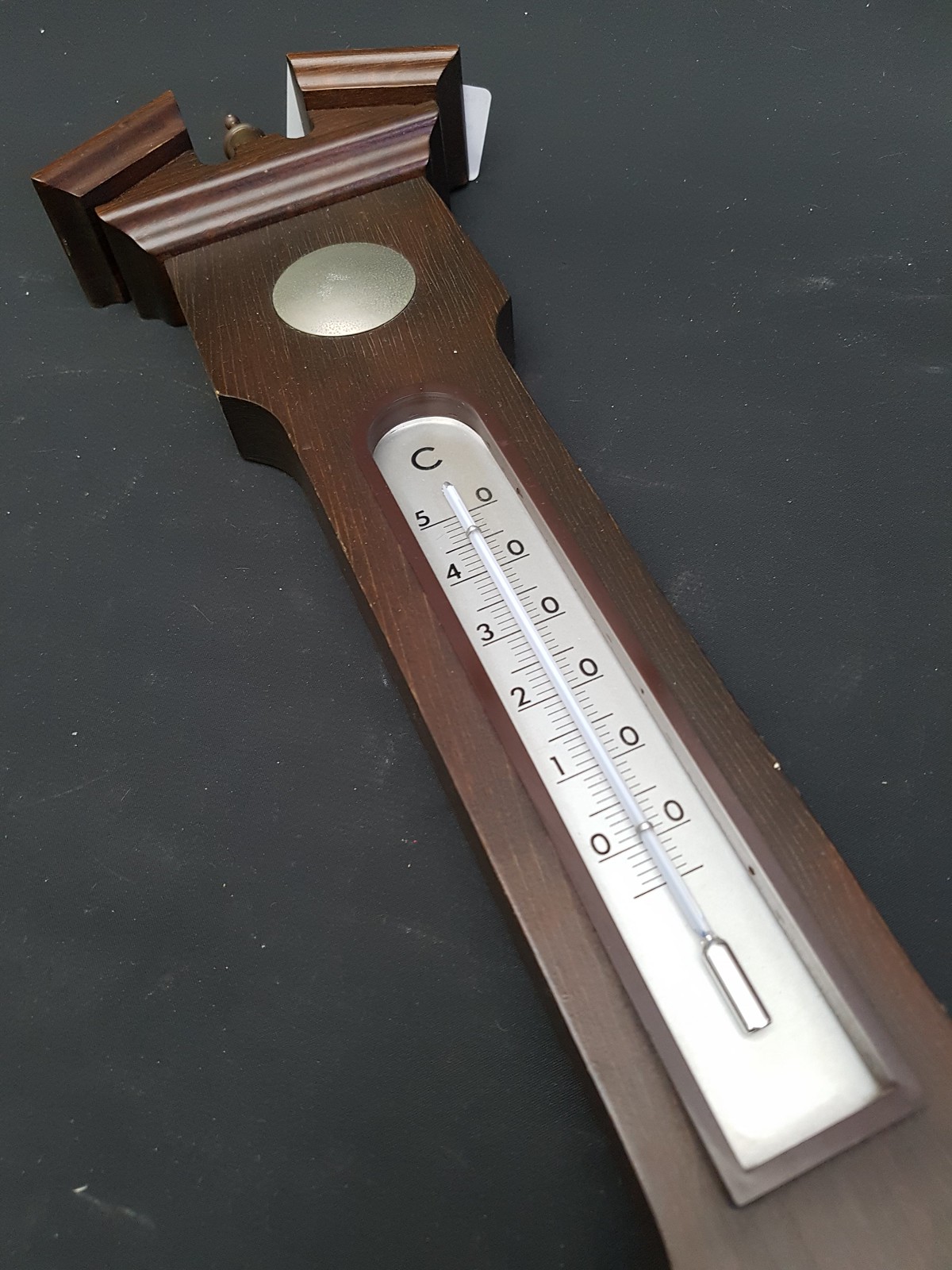The close-up image showcases a wall-mounted temperature gauge encased in a wooden enclosure, distinctively crafted to resemble a small tower. The rich chestnut hue of the wood contrasts elegantly with the dark gray surface on which the gauge is mounted. The temperature gauge has a silvery background, with its temperature scale marked in degrees Celsius. The scale ranges from below zero up to five degrees, with numerals positioned horizontally along the scale to indicate the readings. The letter "C" at the top of the scale confirms the unit of measurement as Celsius.